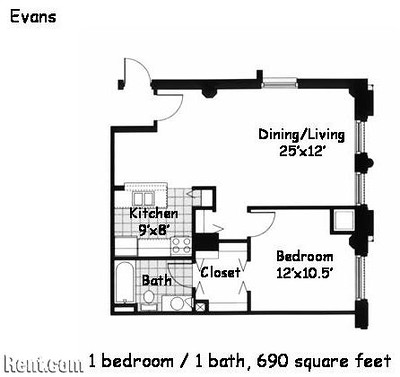This image captures a detailed black-and-white overhead layout of an apartment floor plan set against a white background. The top-left corner features the name "Evans" in bold black letters. A watermark in the bottom-left corner reads "rent.com" in white text.

The layout begins with a door in the top-left section, leading into the apartment. From there, two doors open into a dining/living room area marked with measurements of 25 by 12 feet. Moving to the bottom-right side, the bedroom is outlined with dimensions of 12 by 10.5 feet. Adjacent to the bedroom, on the immediate left, is a closet that offers access to the bathroom located in the bottom-left corner of the plan.

Centrally positioned on the left side, just above the bathroom, is the kitchen, measuring 9 by 8 feet. The overall layout of the apartment is succinctly summarized at the bottom of the image, indicating it is a one-bedroom, one-bathroom unit with a total area of 690 square feet.